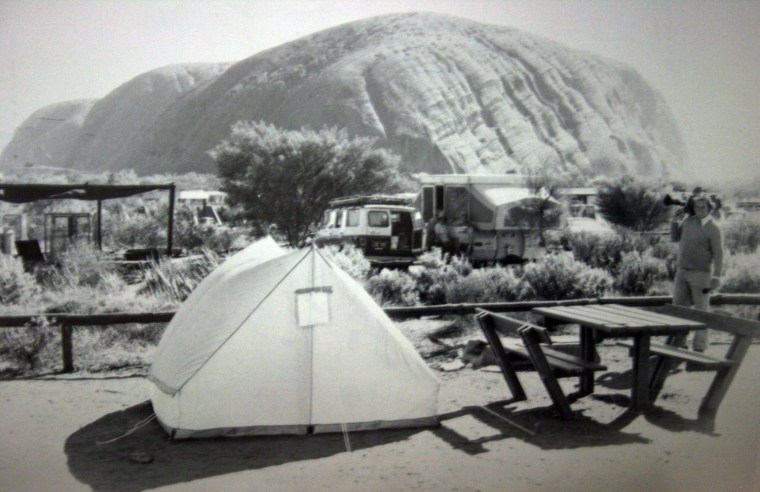This black-and-white photograph, likely from the 1960s or 70s, depicts a campsite set against a vast, arid landscape dominated by a large rocky mountain, possibly Ayers Rock. In the immediate foreground, a light-colored tent, which could accommodate three to four people, is pitched next to a picnic table. Adjacent to the table stands a man wearing a long-sleeve shirt with a white collared shirt underneath, long pants, and holding a camera over his shoulder. The mid-ground reveals elements of a camping community with several RVs, camper trailers, and possibly a shelter among sparse vegetation. Despite the arid setting, plants dot the mid-ground, contributing to the desolate yet lively ambiance of the campsite.